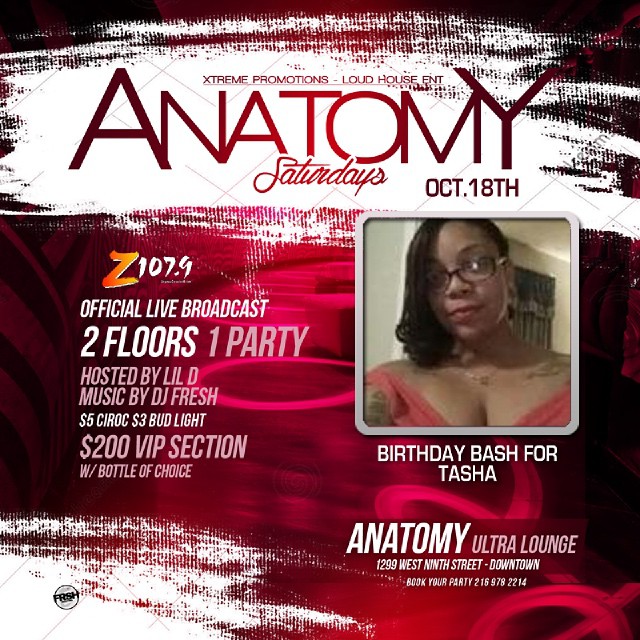This vibrant promotional poster for "Anatomy Saturdays" on October 18th draws attention with its dynamic red and white background featuring swirling and scratched-off designs. At the top, the central title "ANATOMY" is written in bold, stylized lettering transitioning from dark blackish red to bright red and back, flanked by smaller text reading "Extreme Promotions," "Loud House Entertainment," and "ANATOMY SATURDAYS OCT. 18th." The left side of the poster details event information with text announcing "Z107.9 Official Live Broadcast," "Two Floors, One Party hosted by Lil D," "Music by DJ Fresh," "$5 Ciroc," "$3 Bud Light," and "$200 VIP Section with Bottle of Choice." On the right side, a photo of a young African American woman named Tasha is prominently displayed within a white square frame. She has dark, shoulder-length curly hair, wears glasses, a coral dress, a dainty necklace, and showcases tattoos on her arm and shoulder. Beneath her picture, the text reads "Birthday Bash for Tasha," followed by "Anatomy Ultra Lounge, 1299 West 9th Street, Downtown," and "Book Your Party, 216-978-2214." The overall aesthetic of the poster is visually arresting, with its main red hues and contrasting white elements highlighting the essential details.